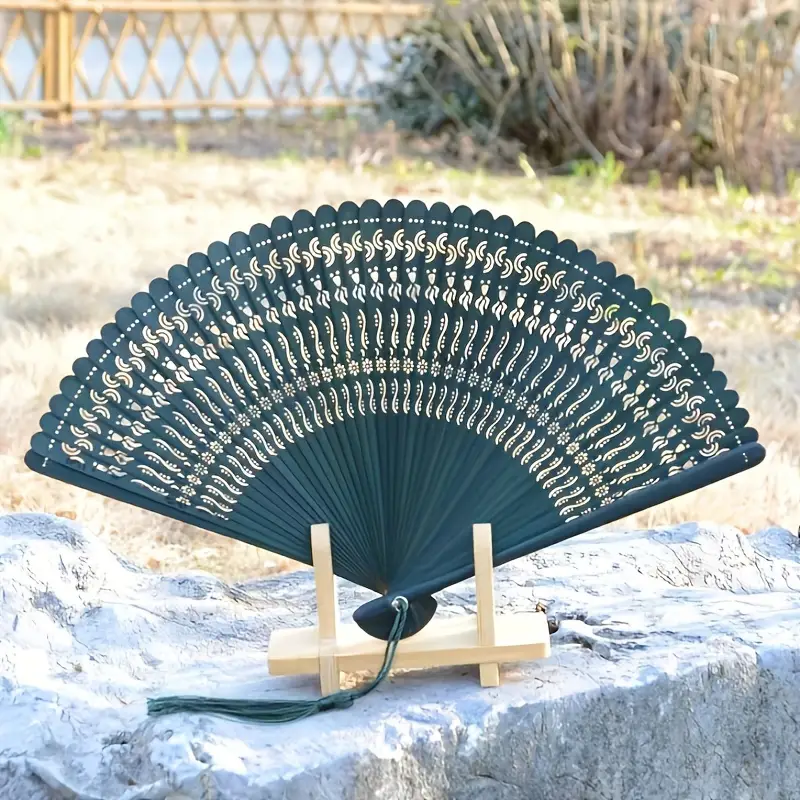The image showcases a hand fan, fully splayed open, situated outdoors on a stone slab. The fan displays a gradient of dark blue to black hues with hints of teal, and it features intricate swirl and flower patterns on its upper portion while the lower section remains a solid bluish-teal. A teal tassel adorns the bottom of the fan. It rests elegantly on a simple wooden holder, likely made of pine or balsa, with its arms supporting the fan on either side. The background, though out of focus, reveals a grassy scrubland with some bushes, a fence, and a distant waterway, all bathed in natural sunlight.